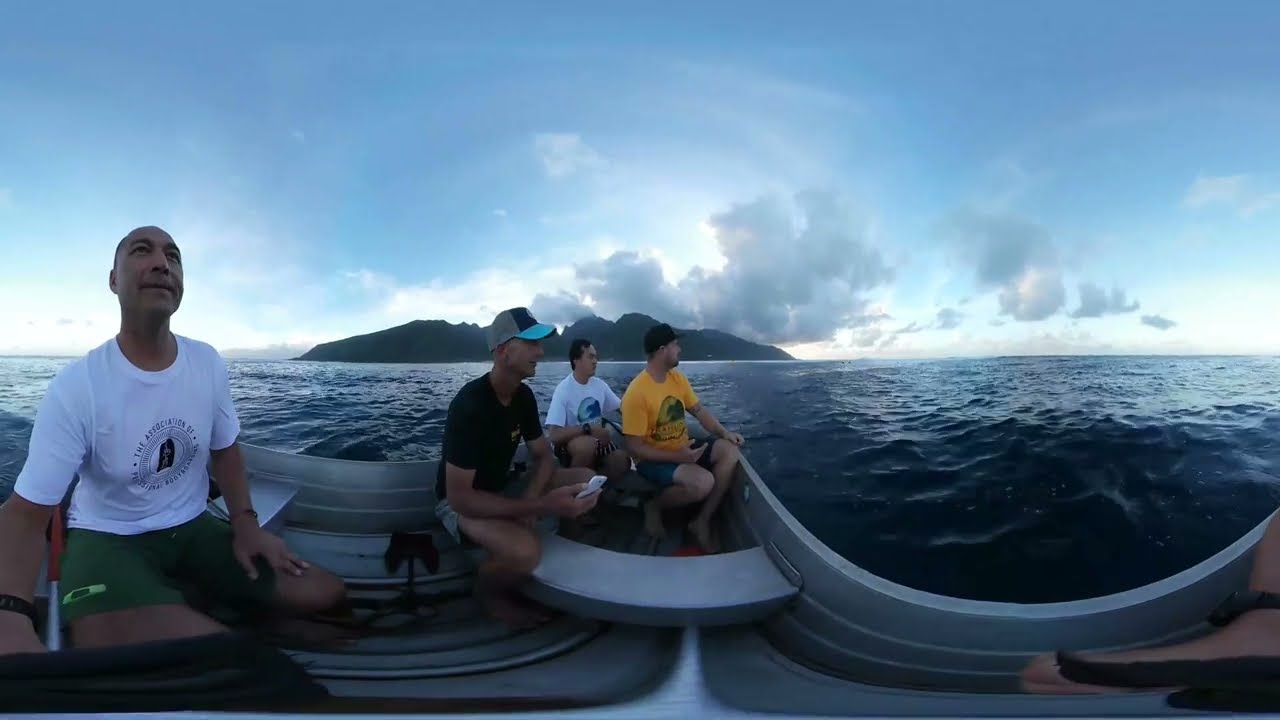The image depicts four men boating on the water during an overcast sunset, captured with a double fish-eye lens that distorts the boat into curved semicircles. The men, dressed in t-shirts and shorts, are arranged seated in the boat, looking off to the right. The man on the left has a bald head and wears a white t-shirt with green shorts. To his right, one man dons a black t-shirt with tan shorts and a blue or green hat, another wears a yellow shirt with blue shorts and a dark hat, and the fourth man, directly behind, is clad in a white t-shirt with a green circle emblem and potentially red and white shorts. The water around the boat appears dark and shadowed, transitioning to lighter shades of gray as it moves away from the boat, reflecting the impending dusk. The sky is deep blue with patches of clouds obscuring the sun, and a rocky shoreline rises in the background to the left. Additionally, an arm of another person can be seen at the far right, indicating the presence of more individuals just outside the frame.